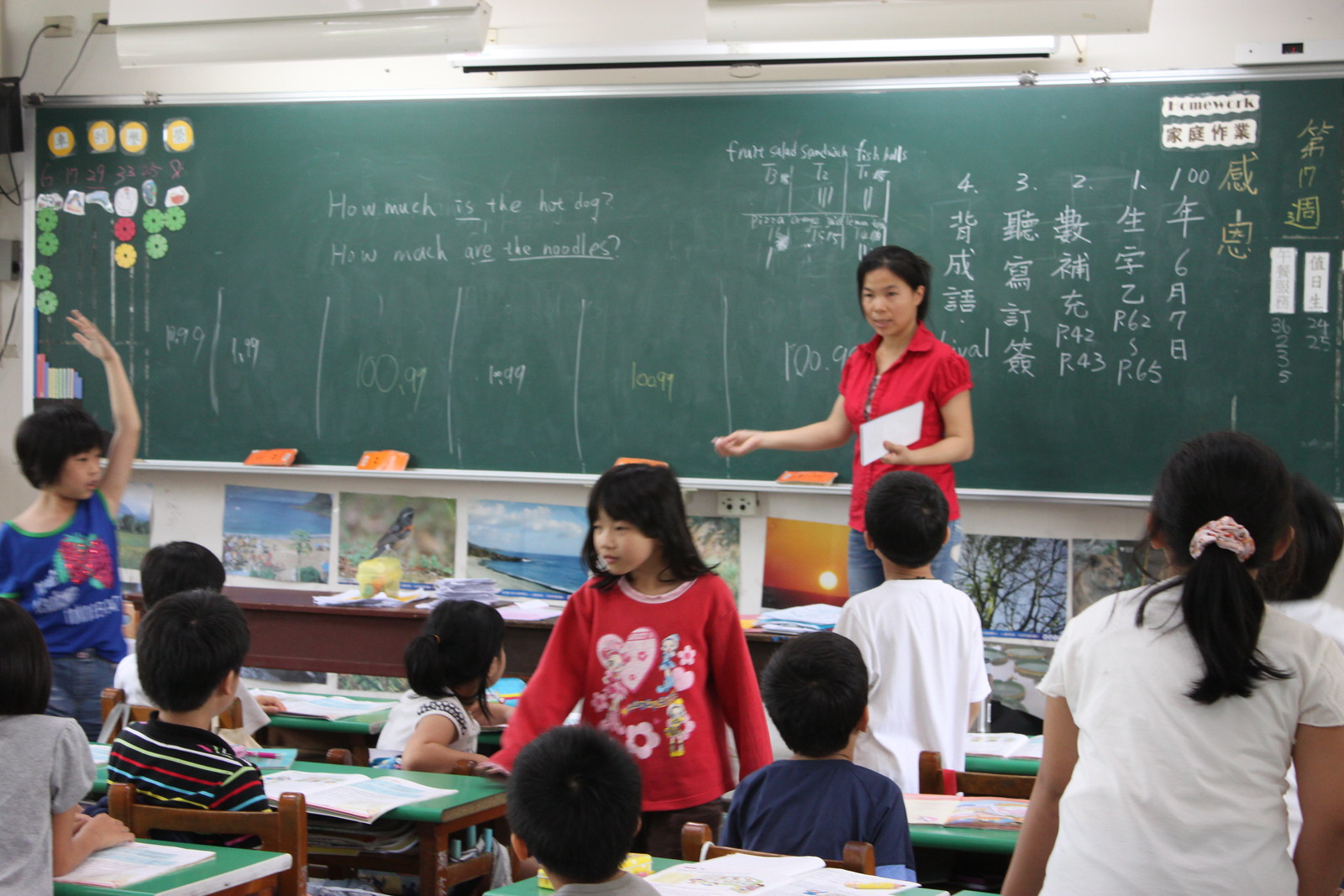In a brightly lit classroom in China, an Oriental teacher stands at a green chalkboard that spans the length of the wall. She is wearing a short-sleeved, red button-down blouse and blue jeans, and she holds a piece of paper in her left hand. The chalkboard displays a mix of English phrases and Oriental characters, with some writing labeled one, two, three, and four from right to left and other parts using both white and yellow chalk. 

Underneath the chalkboard, a row of pictures depicting various scenes adds color to the room. Around 10-12 children, a mix of genders, sit at desks with green surfaces, their backs turned towards the viewer and their eyes focused on the teacher and the board. The children, some with long hair and others with short black hair, are engaged in their workbooks and occasionally raise their hands. The overall atmosphere suggests a lesson focused on both English and their native language.